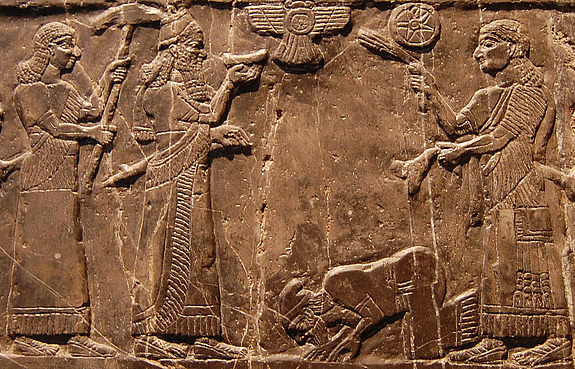This photograph captures a detailed clay-brown mural with intricate carvings depicting a scene reminiscent of ancient Sumerian art. The mural features four engraved figures on a stone-like wall. On the left, two men are standing; the man farthest left holds a giant hammer or a sickle, while the man next to him appears to be holding a piece of bread or a plate. On the right side of the mural, another man stands and faces left, holding two objects that resemble a bushel of weeds or tools. Between the standing figures on the right is a man on his hands and knees with his head bowed to the ground, appearing to beg. Above the figures, there is a medallion and a symbolic bird, possibly resembling an eagle, adding to the antiquated aesthetic. This scene is carved with high detail, evoking the artistic styles of ancient civilizations, albeit neither definitively Egyptian nor clearly identifiable from the image alone.